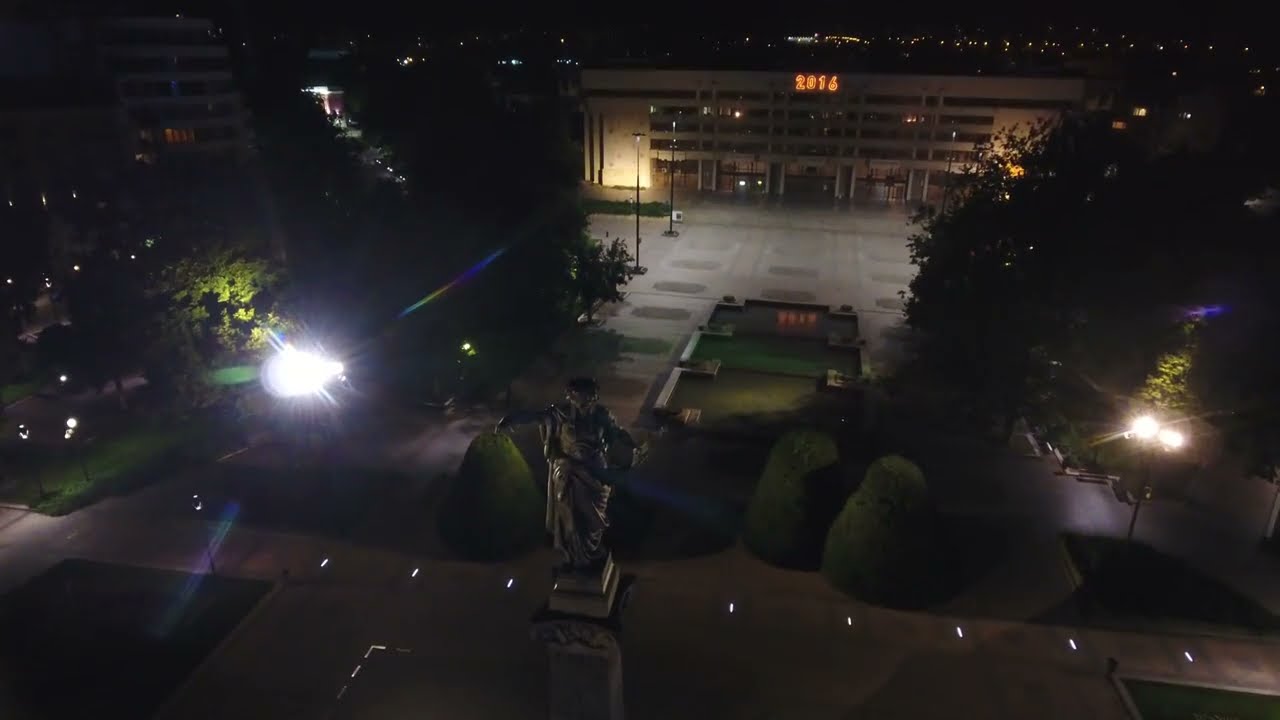The nighttime aerial photograph captures the tranquil atmosphere of a large, empty courtyard on a college campus. The photo, likely taken from a drone, offers a bird’s-eye view of a distinctly multi-story building, presumably a campus library, with the year "2016" illuminated prominently on its facade, potentially indicating the year the photo was taken. At the center bottom of the image, a statue of a woman adorned in a Greco-Roman style toga stands amid the courtyard. She is surrounded by a sprawling stone pathway embedded with lights that illuminate the scene, creating a starburst effect particularly noticeable near a bright white streetlight to the statue's left. The courtyard features a green grass median that possibly doubles as reflective ponds, adding a touch of verdant beauty to the stony expanse. In the background, city lights twinkle, further enhancing the aura of this serene nocturnal landscape.